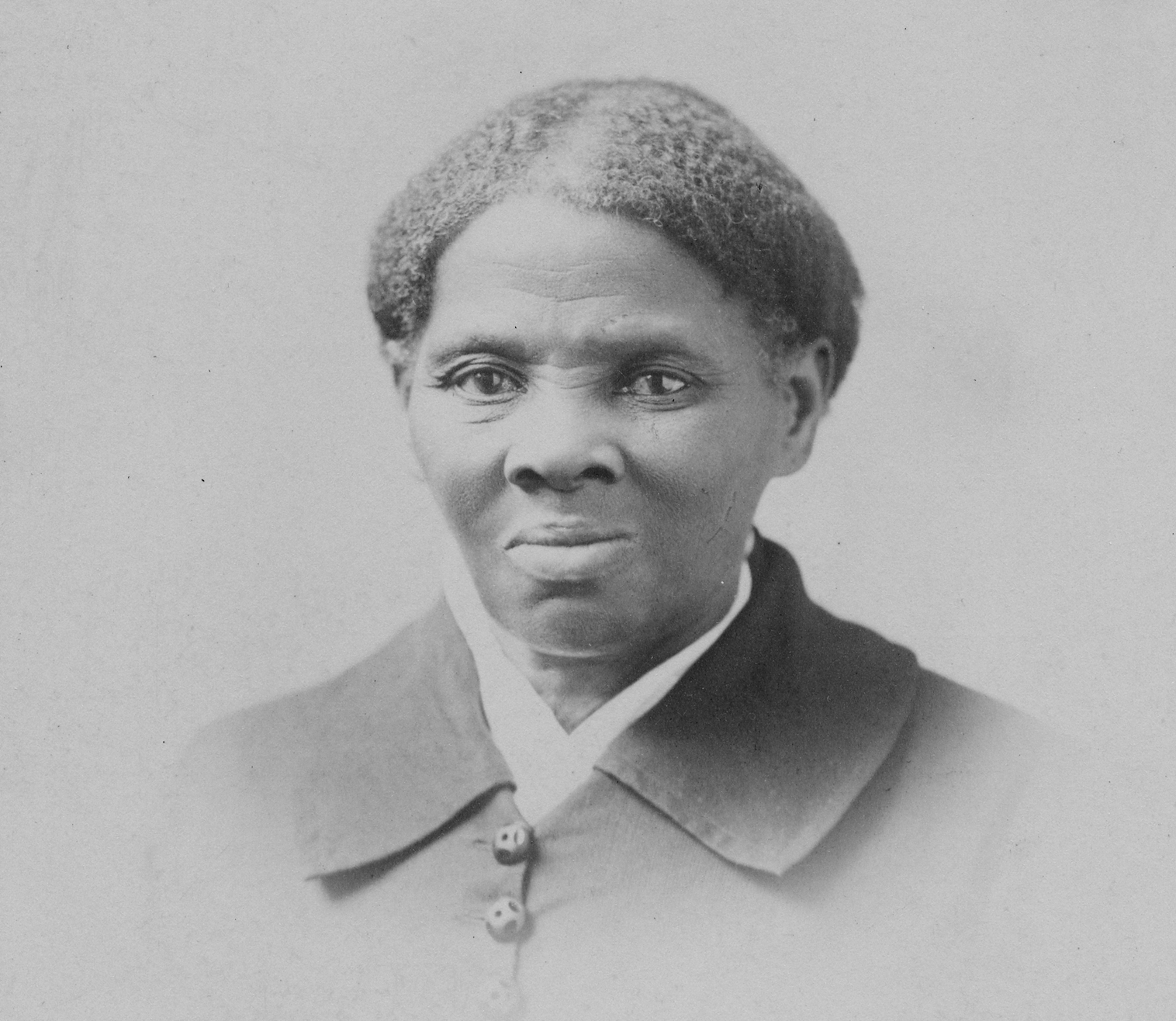This black and white photograph is a portrait of a black woman who exudes a sense of sternness and seriousness. The image, which appears very old and has faded around the edges, draws primary focus to her face, capturing fine details such as the wrinkles around her eyes and the lines between her furrowed brows. Her gaze is direct, and her expression is neutral, neither smiling nor angry. Her short, natural, and matted hair is pulled back, revealing her face clearly. She is dressed in a white collared undershirt and a darker jacket with buttons visible down the front. The coat appears practical, with no adornments like jewelry or makeup, highlighting the simplicity of her attire. The background is an unadorned gray, further emphasizing the solitary figure in the photograph.